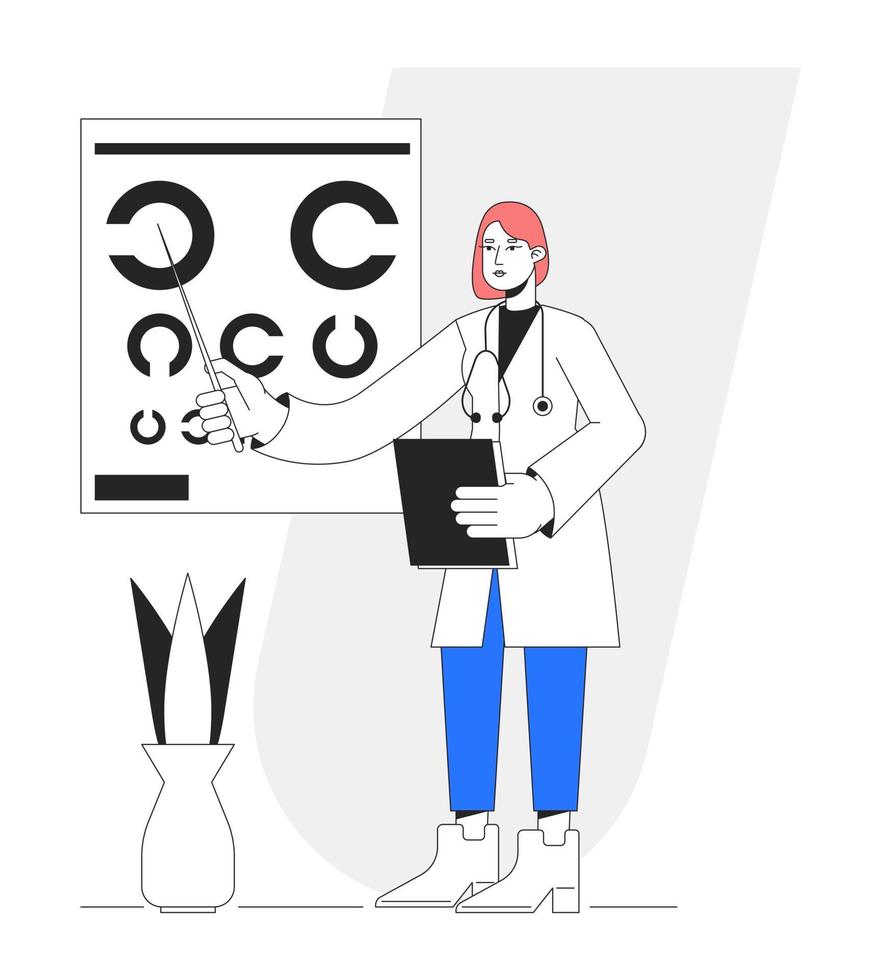This digital illustration is a detailed line drawing featuring a stylized eye doctor, likely an ophthalmologist or optometrist, set against a simplistic white background with a subtle gray half-oval shape. The doctor, a woman with red hair and unusually small head, is adorned in a white lab coat over a black shirt, blue scrubs, and white boots. A stethoscope is draped around her neck. In one hand, she holds a black clipboard or pamphlet, while the other wields a pointer directed at an eye chart. This eye chart, a prominent feature in the image, consists solely of the letter 'C' in various sizes and orientations, mimicking a typical optometric chart. Beside her, on the floor, is a black and white planter holding three large leaves, adding a touch of organic element to the clinical setting. The overall composition remains flat and monochromatic, emphasizing the scene with tonal contrasts.